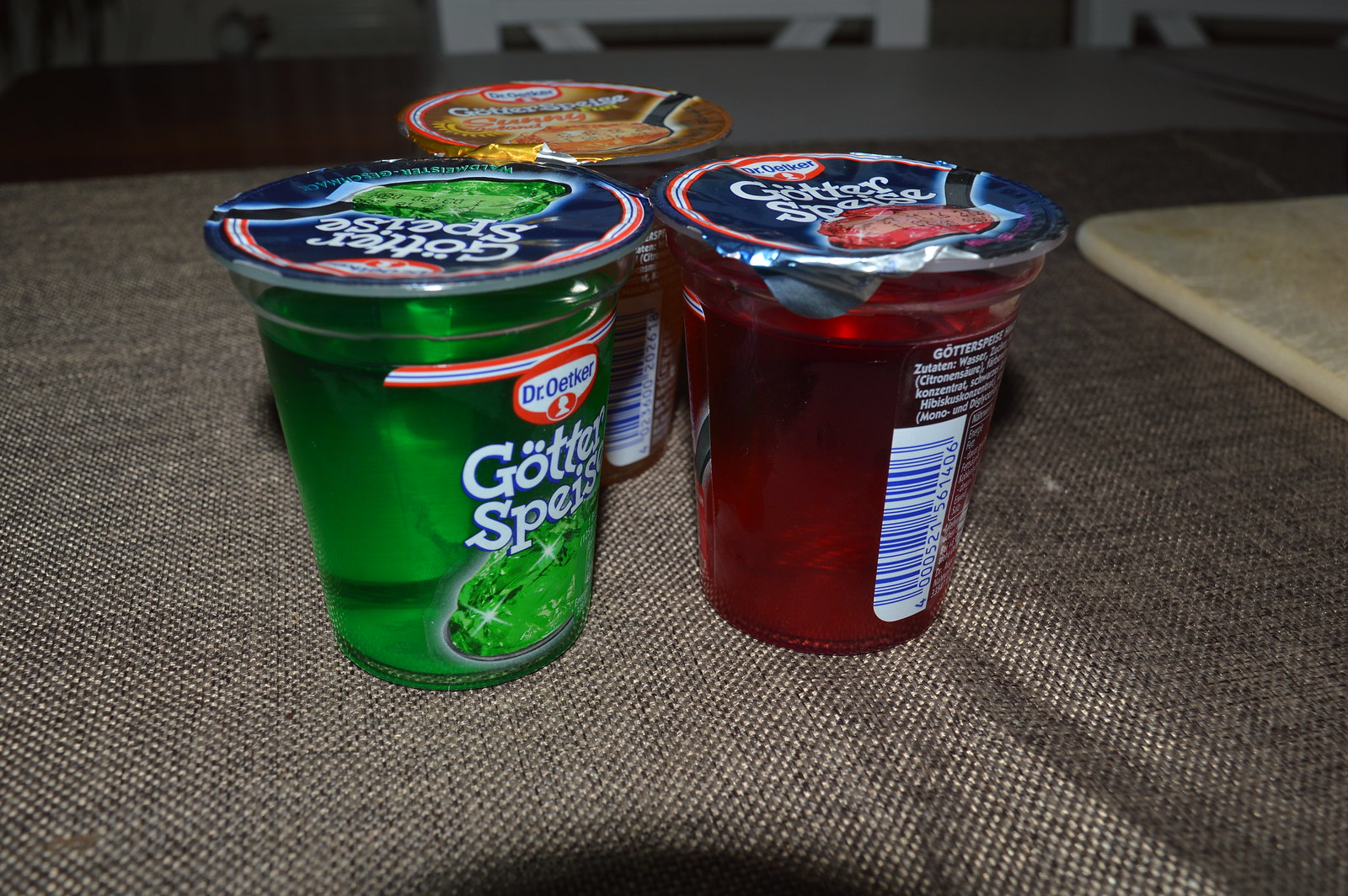The close-up photograph captures three clear, plastic containers of gelatin dessert, each sealed with a foil lid. Arranged on a wooden table draped with a slightly wrinkled, grayish-brown tweed tablecloth, the containers come in three vibrant colors: green, red, and orange—likely indicating lime, cherry, and orange flavors, respectively. Each lid features a dark navy background with red and white edging, showcasing images of the corresponding flavors, and the name "Dr. Oetker" along with "Götterspeise" written in German. A light-colored cutting board is positioned off to the side, and a counter can be seen in the background, adding a touch of kitchen ambiance to the scene. These details highlight the simple yet inviting setup, focusing on the colorful, inviting gelatin cups ready to be enjoyed.